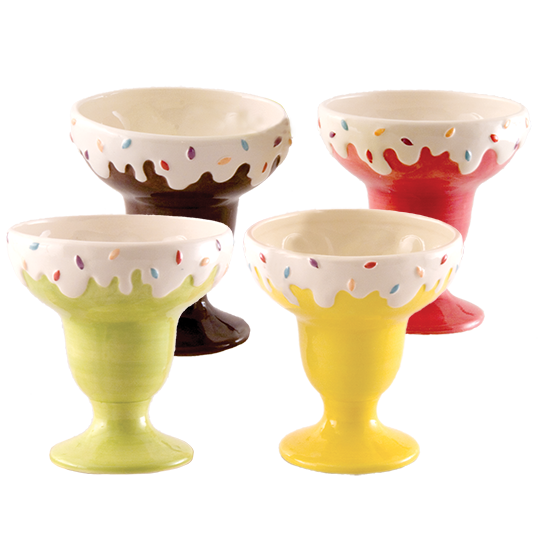The image displays four ice cream cups, each with a unique color and a decorative topping. The cups are arranged in a square against a white background. The bottom left cup is light green, the bottom right cup is yellow, the top left cup is brown, and the top right cup is pink. Each cup features a white, dripping decoration at the top, resembling melted white chocolate or frosting, adorned with an assortment of multicolored sprinkles in shades of tan, blue, red, purple, light blue, and light pink. The cups appear to be made of plastic, though they could also be ceramic. The overall design of the cups is uniform, with a round base that widens at the top. The sprinkles and dripping white decoration add a playful and vibrant touch to the otherwise simple design.